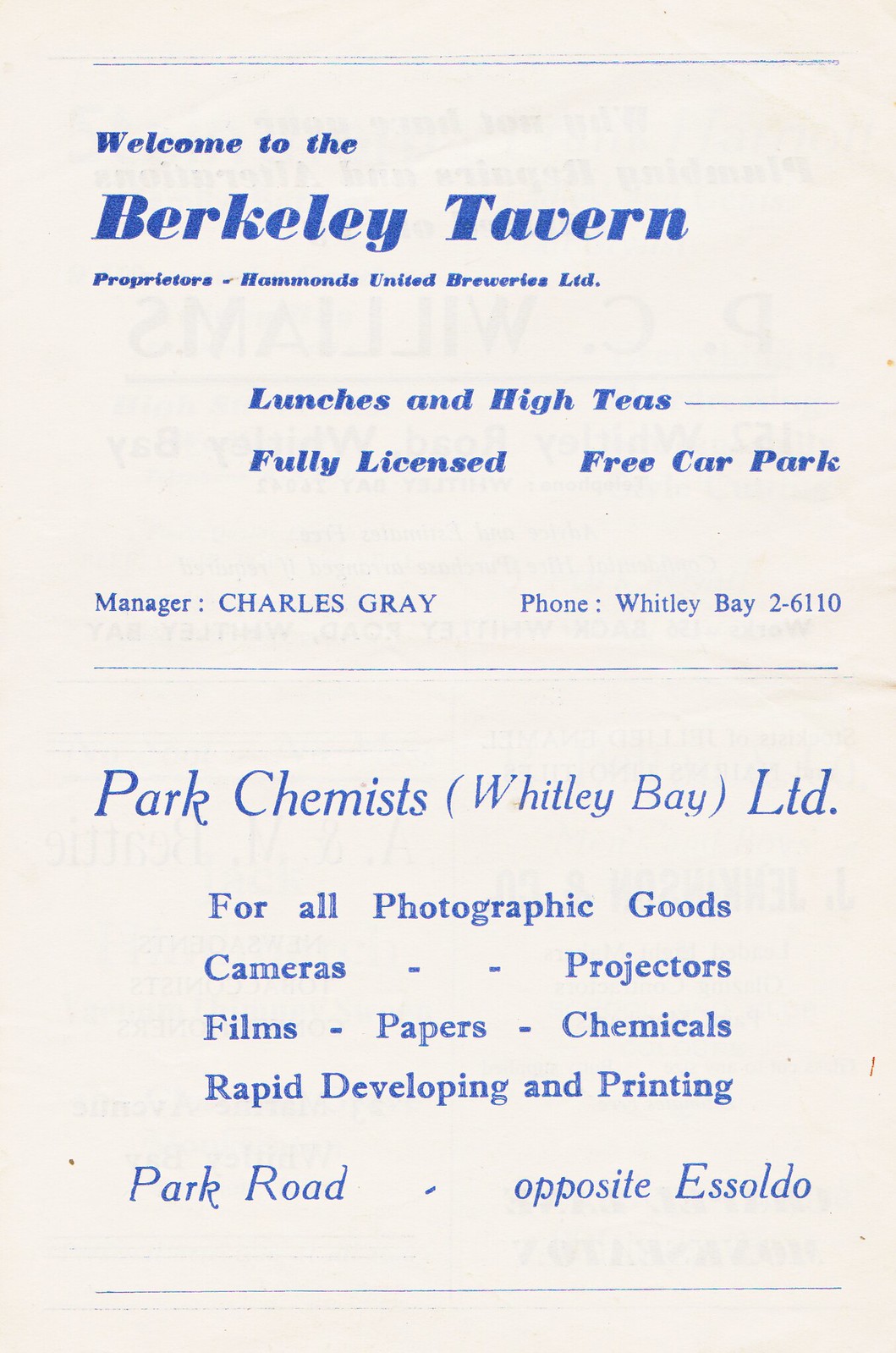The image is a tall rectangular pamphlet with a very pale off-white background. On the top and bottom, there are thin horizontal blue lines. The largest text at the top reads in bold blue letters, "Welcome to the Berkeley Tavern." Below that, in smaller blue text, it states, "Proprietors Hammond's United Breweries Limited." Following this, it mentions "Lunches and High Teas, Fully Licensed, Free Car Park." The manager is listed as "Charles Gray," with the contact information "Phone: Whitley Bay 2-6110." After a blue line break, the pamphlet details services provided by "Park Chemist (Whitley Bay) Limited" which includes "Photographic Goods, Cameras, Projectors, Films, Papers, Chemicals, Rapid Developing, and Printing." The location is given as "Park Road, Opposite Esoldo."